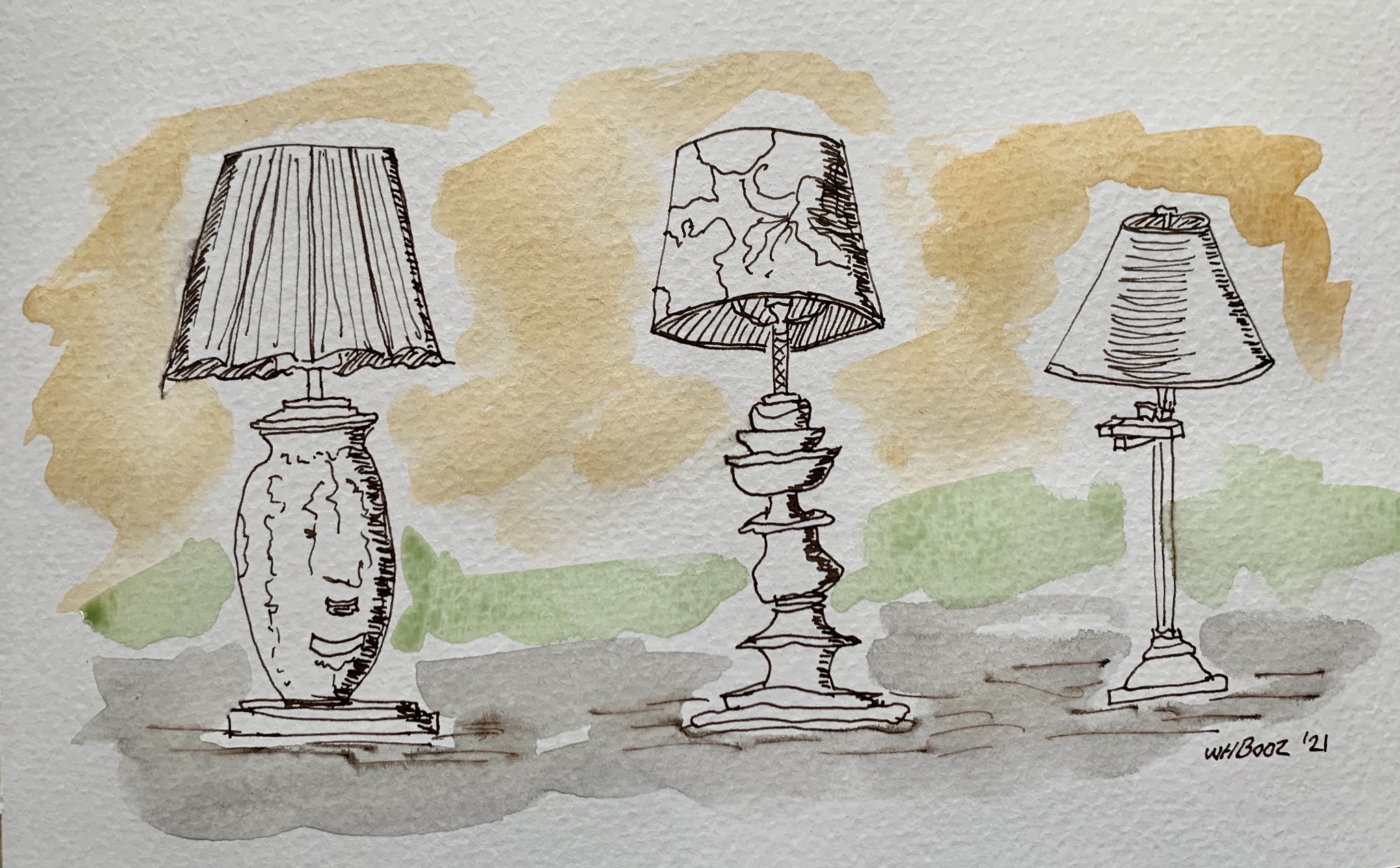This image is a detailed watercolor art piece on white paper, depicting three uniquely styled table lamps drawn in black pen. Each lamp features distinct characteristics and details outlined and shaded with black ink. The lamp on the far left has a round base that resembles a face, complemented by a pleated lampshade. The middle lamp boasts a multi-layered base with a lampshade that appears to have a map pattern. The lamp on the right is the smallest, with a simple, flat lampshade and a long, slender handle. The background of the painting is richly colored with gray watercolor around the bases, green around the centers, and a yellowish-golden hue at the tops, transitioning to a subtle orange. The artwork is signed “WHBooz21” in black ink in the lower right corner.